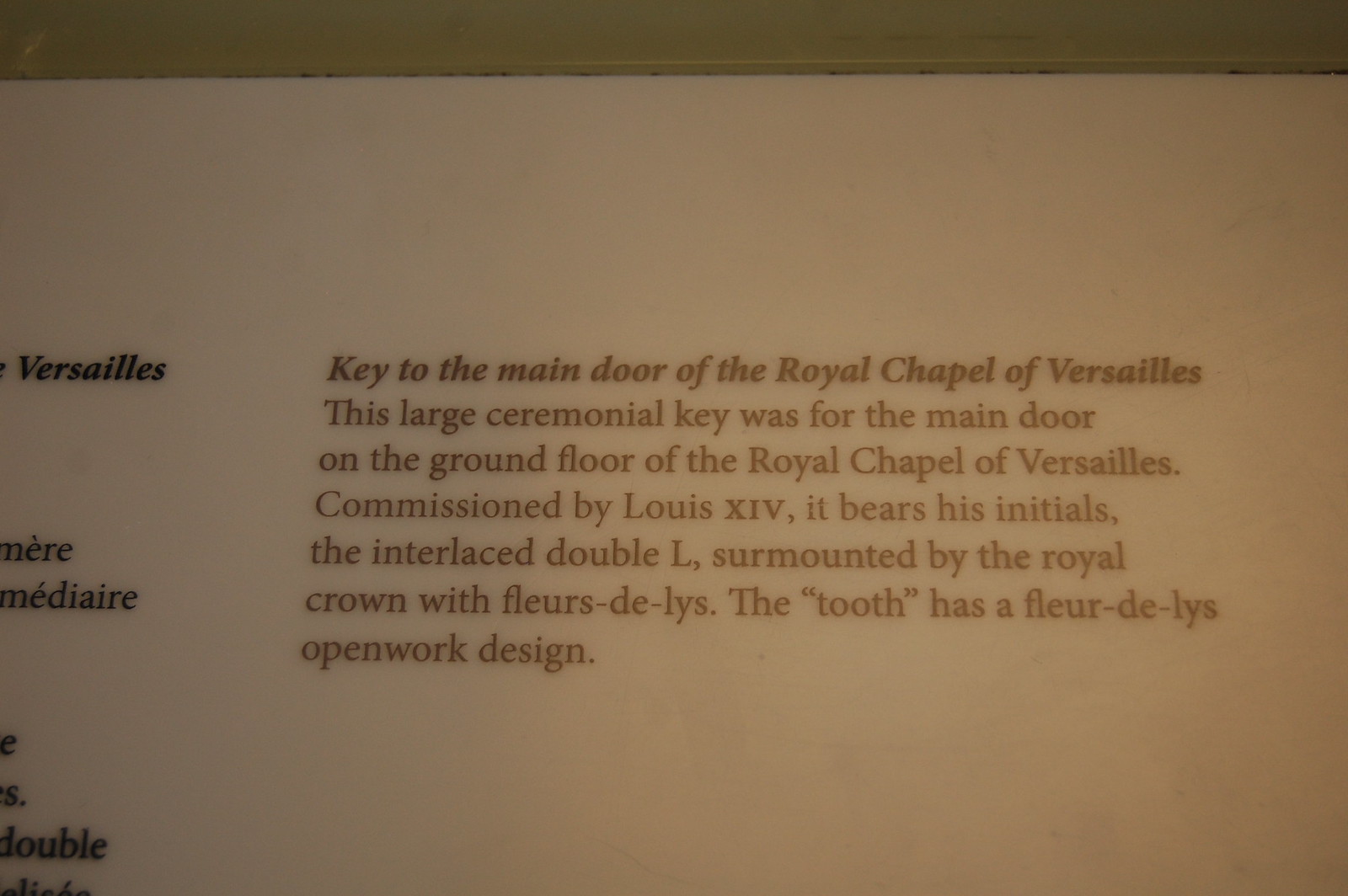This horizontal, rectangular color photograph is a close-up of an informational tour sign about a ceremonial key, taken in dim light, making the image dark and the text slightly hard to read. The white background of the sign has brown text, while on the left side, some black text can be partially seen with the word "Versailles" visible. The highlighted paragraph in brown reads: "Key to the main door of the Royal Chapel of Versailles. This large ceremonial key was for the main door on the ground floor of the Royal Chapel of Versailles. Commissioned by Louis XIV, it bears his initials, the interlaced double L, surmounted by the royal crown with fleur-de-lis. The tooth has a fleur-de-lis openwork design." At the top of the page, a darker border suggests it is resting on a dark surface, surrounded by the darkness of the room.